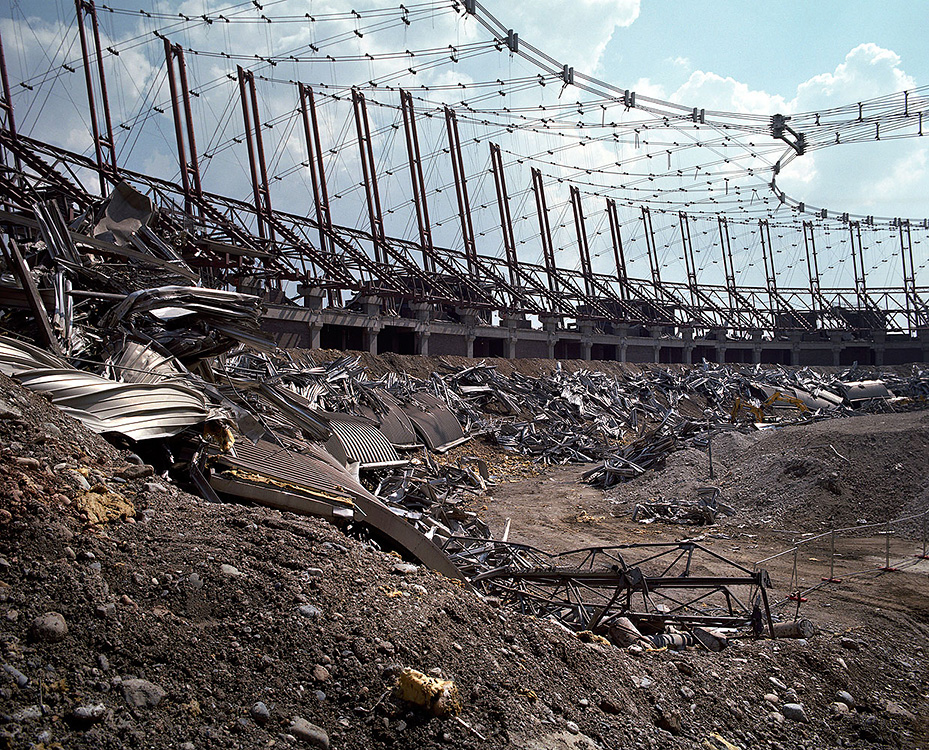The image captures an expansive outdoor scene on a clear, pleasant day with a light blue sky dotted with white clouds. Dominating the scene is a large, circular pit filled with piles of scrap metal, dirt, rocks, and debris, likely from a deconstructed building or an abandoned stadium. Surrounding the pit is a tall fence, reinforced with netting that partially covers its expanse. Pieces of dark, black-colored metal define the perimeter, possibly remnants of the stadium's infrastructure. Scattered around the area are upturned furniture, wooden shelving, and twisted structures, hinting at a chaotic abandonment. Metal poles and a silver structure overhead suggest these may have been parts of an awning or stadium covering. A dirt roadway runs along the bottom edge of the frame, further emphasizing the desolate, scrapyard-like atmosphere of the scene.